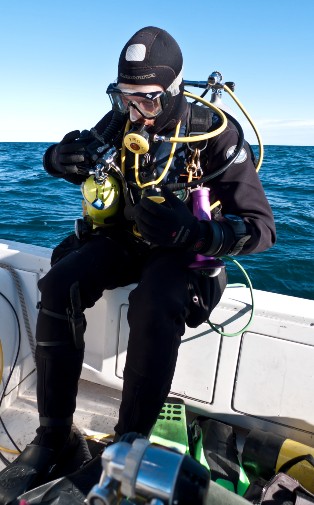In this outdoor daytime photograph, we see a Caucasian male diver in the center, preparing to enter the ocean from the edge of a white boat. The diver is dressed in a slightly loose-fitting, all-black wetsuit, complete with black fins and a diving mask with a yellow regulator in his mouth. He is equipped with two yellow air tanks—one on his back connected by airlines to his breathing apparatus, and another smaller tank under his right arm. The diver's head is bent down, possibly checking the pressure gauge on the smaller tank. Additional gear includes a flashlight on his waist belt and a knife strapped to his right leg. The diver's suit features a square silver patch on the top of his head, although its details are indiscernible. The deck of the boat is scattered with various equipment, including a possible fishing rod, a pinkish tube, and a silver fisherman's reel. Behind the diver, the ocean extends into the horizon, transitioning from deep blue water to a lighter blue sky that turns nearly white where it meets the sea.